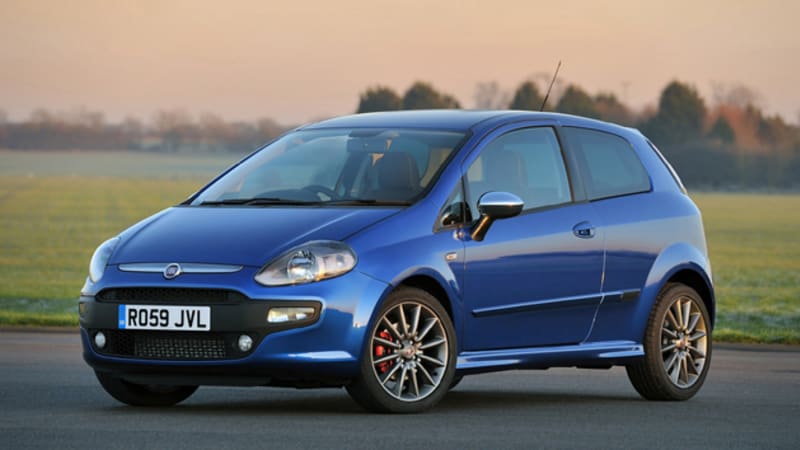This photograph captures a small, bright blue, two-door hatchback, potentially a Fiat, parked on a smooth pavement. The vehicle is accented with silver rims and black tires, a silver front badge, and a white license plate reading "R059 JVL." An antenna is visible at the rear of the car. The right headlight is clearly seen, while the left is partially obscured. The backdrop features a flat, grassy field transitioning into a tree-lined horizon with green and orange foliage. The sky above is an evocative blend of peach and gray hues. There are no people present in or near the car, emphasizing its solitary presence against the natural setting.